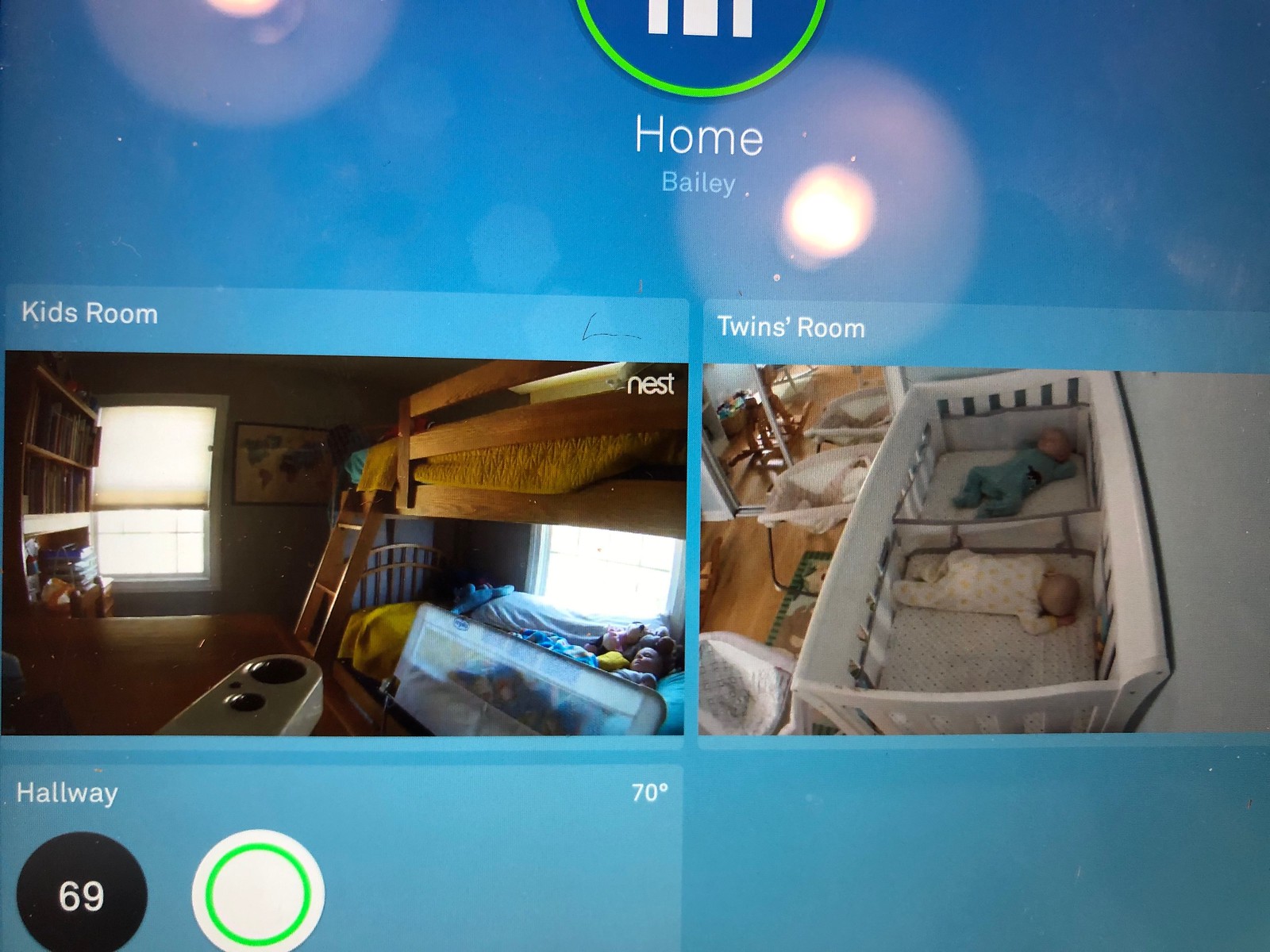The image appears to be a composite view from a home surveillance system. The background is a solid blue screen with the heading "Home" in white text at the top, followed by "Bailey" in blue text. Below this header, the screen is divided into two sections, each showcasing a different room.

The left section is labeled "Kids Room" in white text. The live feed reveals a dimly lit room with bunk beds. The top bunk is accessible via a ladder, and two windows are visible, though they allow limited natural light into the room. Beneath the "Kids Room" picture, there is additional information: it mentions "Hallway" and indicates a temperature of "70 degrees." Adjacent to the hallway label is a black circle with "69" written in white text inside it, accompanied by a white circle enclosing a smaller green circle.

The right section is labeled "Twins Room" in white text. The live feed shows a crib with a central divider, accommodating two infants. Both babies are lying down, each in their own separate half of the crib, ensuring they have distinct spaces within the shared crib.

This detailed setup assists in monitoring different areas within the home, providing specific information about each room's conditions and current occupants.